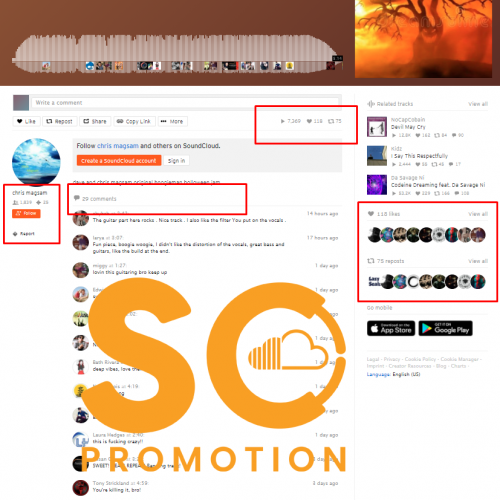The image depicts a screenshot from what appears to be a SoundCloud webpage, partially obscured by a large overlay with the text "SO Promotion" in bold, prominent letters. At the top of the page, there is a Halloween-themed image featuring a haunting tree with a face resembling a jack-o'-lantern carved into its trunk, emitting an eerie orange glow. The tree's smoldering leaves and fiery ambiance add to its sinister appearance. Surrounding this image are indistinct elements, with a noticeable brownish hue.

Towards the center, there's a highlighted interaction section displaying the option to "Write a Comment," accompanied by buttons for "Like," "Post," "Share," and "Copy Link." A significant highlight shows a count of 7,363 likes, indicated by a heart symbol, implying the image's popularity.

In the upper left corner, the user's name, Chris Magnum, is visible, along with a small icon depicting a serene sky scene. Beneath the main image, various user comments are visible, albeit partially zoomed out. One comment mentions "the guitar can't have something," while another user, known as Fast Pirate, is acknowledged. A distinct comment reads, "You're killing it, bro."

On the right side of the page, there are several images resembling CD covers, noted to have garnered 115 likes. The page further promotes mobile accessibility with mentions of the App Store and Google Play, suggesting this is a desktop view of the site. Additionally, the section "Related Tracks" highlights titles such as "Devil May Cry," "The Kids," and "Die Savage."